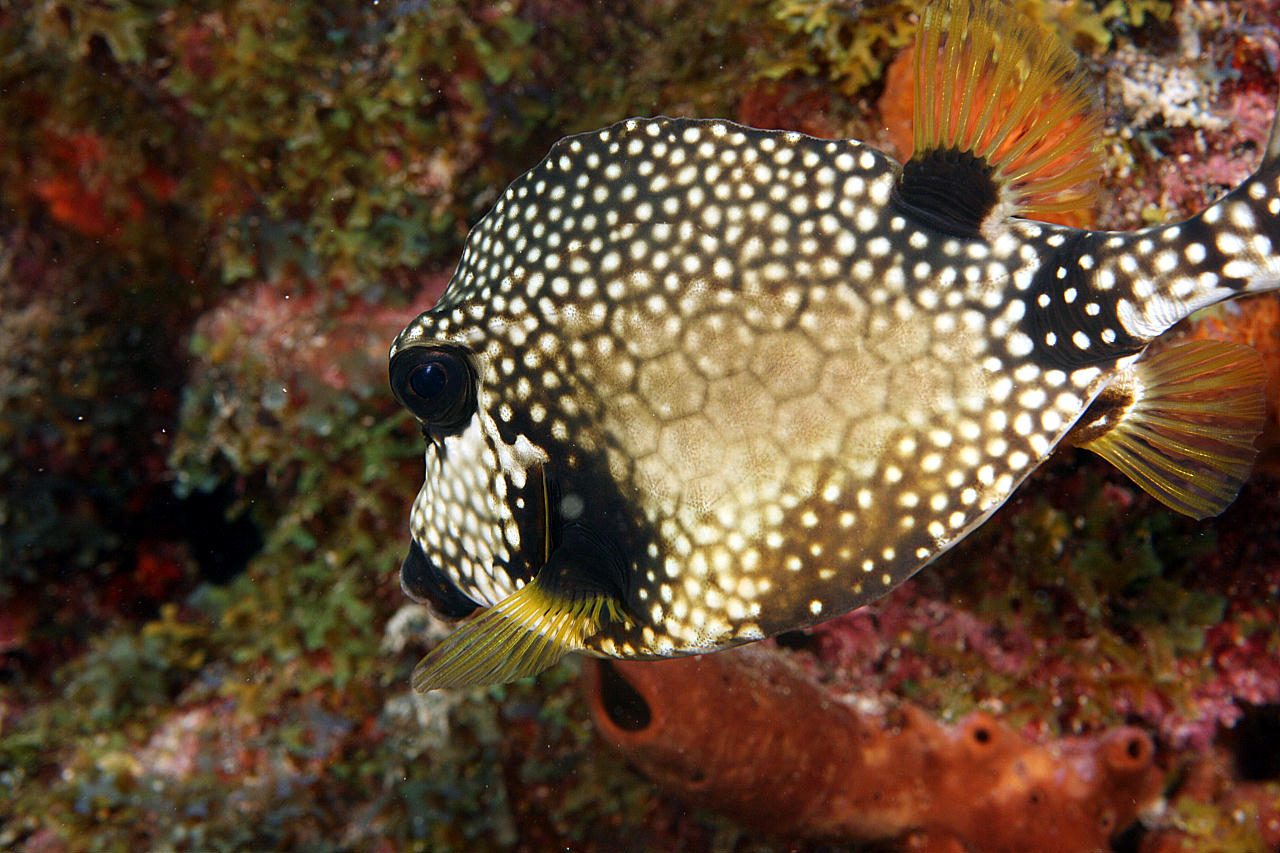This captivating underwater scene features a brightly colored tropical fish prominently displayed in the center. The fish, predominantly black, white, and cream-colored with an intricate pattern of white spots and diagonal markings, has a distinct black mouth and a prominent dark eye positioned center-left. It displays translucent fins on its bottom portion and vibrant yellow spines along its back. The fish spans from the top left to the bottom middle of the image, surrounded by a diverse and vivid coral reef. The reef showcases an array of colors, including blues, greens, pinks, reds, and whites, creating a textured backdrop filled with tubular shapes, holes, and cracks. A hollow piece of red-orange coral stands out beneath the fish, adding to the complexity of the scene. Overall, the image captures a moment of natural beauty, teeming with color and detail, highlighting the fish among the lush coral structures of the ocean.